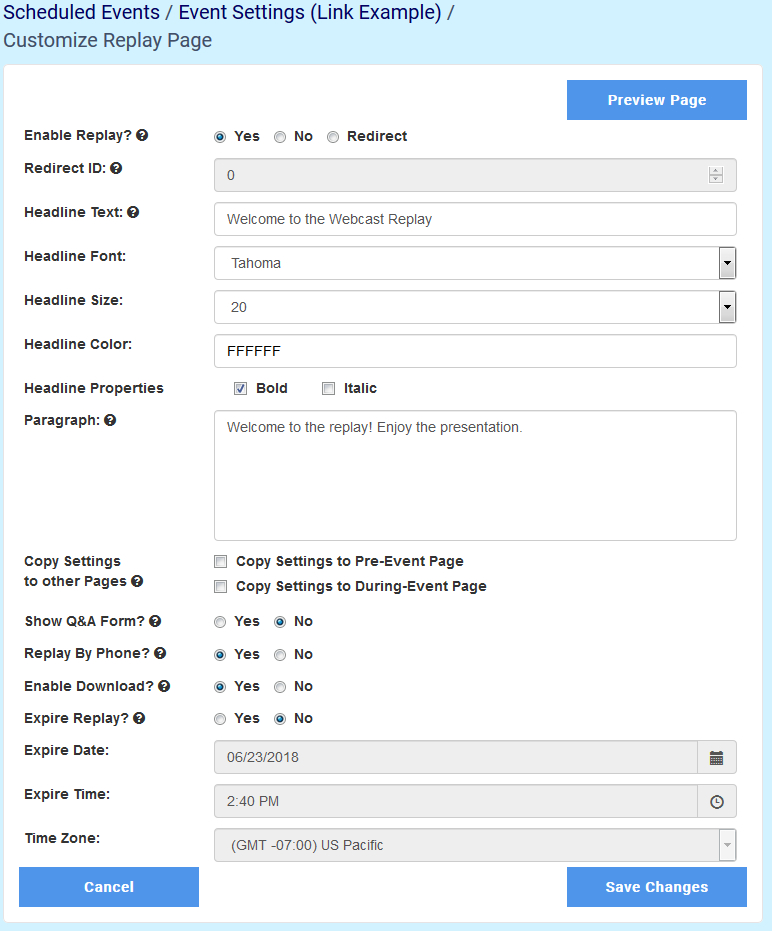This image appears to be a screenshot taken from a web interface, specifically a settings or configuration page for scheduled events. The top of the page displays a header in light bluish-teal color, titled "Scheduled Events / Event Settings".

The majority of the background is white with a few rectangular sections highlighted in blue and grey for easier navigation and emphasis. The left sidebar lists several customizable elements in darker black print, each accompanied by a question mark to indicate additional information is available upon hovering or clicking. These elements include:

- Enable Replay [?]
- Redirect ID [?]
- Headline Text [?]
- Headline Font
- Headline Size
- Headline Color
- Headline Properties
- Paragraph [?]

Below these customizable options, there is a blank space followed by a series of other customizable commands and options, each ending with a question mark:

- Copy Settings to Other Pages [?]
- Show Q&A Form [?]
- Replay by Phone [?]
- Enable Download [?]
- Expire Replay [?]

Under these options, fields are available for entering the expiration date, expiration time, and time zone, but these do not come with question marks. 

Additionally, there are clear buttons for user actions at the bottom of the page. One button is labeled "Cancel" to abandon changes, another labeled "Save Changes" to apply the new settings, and at the top right corner of the page, there is a button labeled "Preview Page" for reviewing how the settings will appear once implemented.